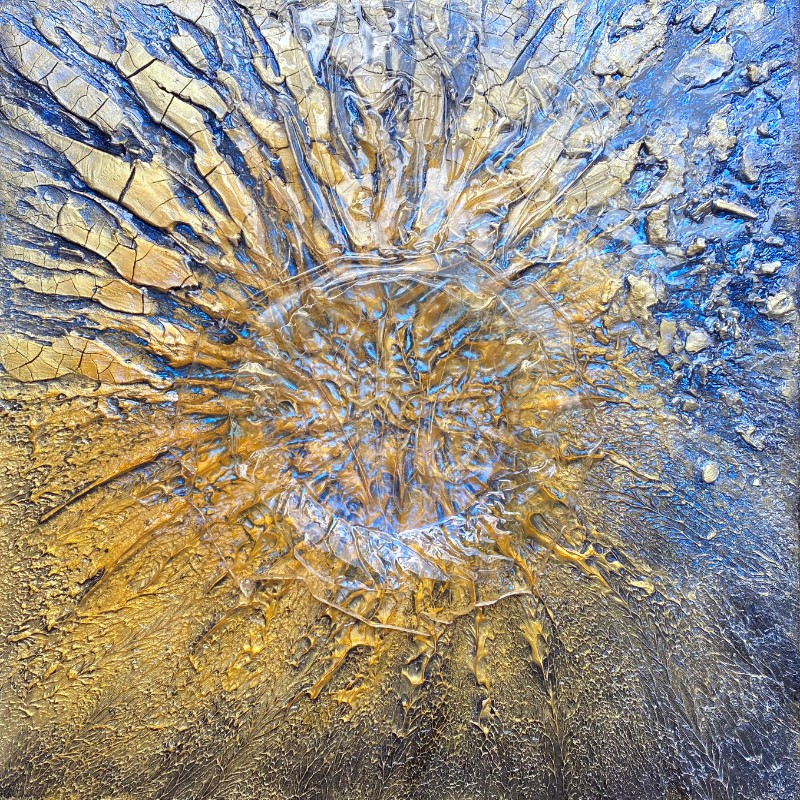The image depicts a textured, almost 3D-like piece of abstract artwork, potentially created with oil pastels. Central to the composition is a circular, raised section resembling the top of a volcano or a radiant sun, highlighted in colors of gold, off-white, and various shades of blue. This central circular form appears to emanate rays or lines that radiate outward, giving it a dynamic, radiant quality. Surrounding this central feature are cracked fragments, possibly of golden and off-white paint, enhancing the textured effect. The background is predominantly blue, ranging from light to dark shades, with splashes and spatter marks that add to the abstract nature of the artwork. There are no organic elements such as animals or people, and no text, focusing entirely on the artistic interplay of colors and textures.